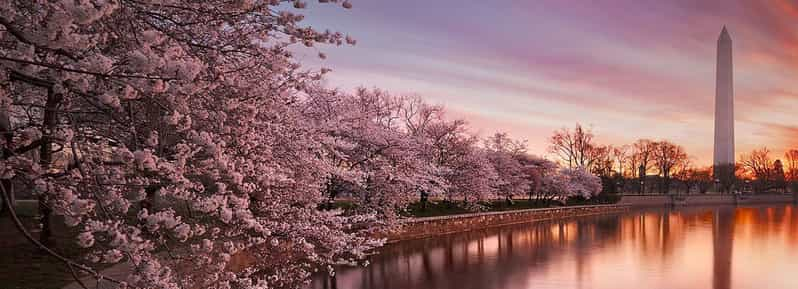The photograph captures a breathtaking view of the Tidal Basin in Washington, D.C., at sunset. The rectangular image reveals the sky transitioning into hues of purple, pink, and orange as the sun sets low on the horizon to the right. The scene is dominated by a body of water encircled by a man-made brick retaining wall that curves from the bottom left towards the center right. Lining this wall is a row of cherry blossom trees in full bloom, their branches adorned with fluffy white and pinkish blossoms, signaling the early days of spring. Further along the shoreline, taller trees are visible, adding depth to the composition. Far in the background stands the Washington Monument, a tall, pencil-shaped structure pointing skyward. The warm tones of the setting sun bathes the landscape in an ethereal golden light, with the clouds reflecting a soft, purplish-orange glow. This image not only marks the iconic beauty of cherry blossoms in peak bloom but also embodies the tranquil yet vibrant atmosphere of D.C.'s National Mall at twilight.